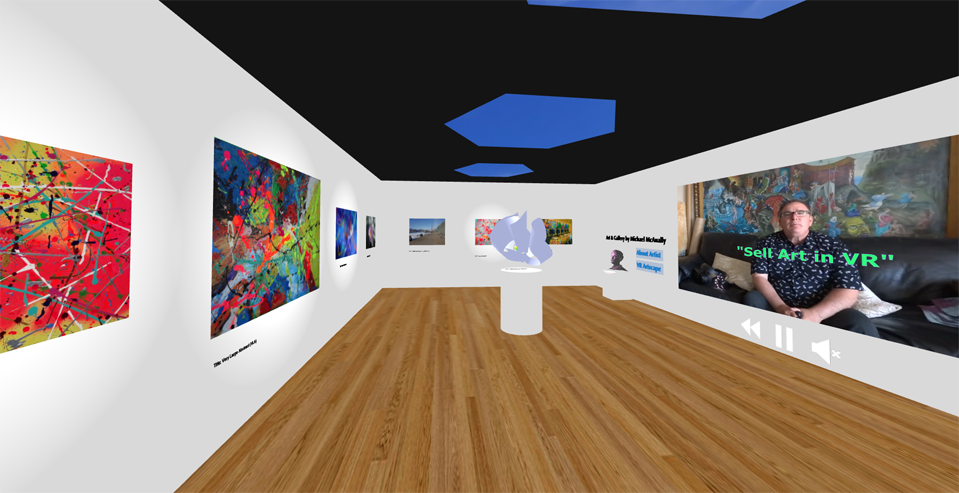The image is a detailed digital screenshot of a 3D-rendered virtual room, designed to represent an art gallery. The room features white walls adorned with various vibrant paintings, some abstract and rich in colors like red, orange, purple, and blue. On the left wall, the painting focused on the extreme left is slightly off-frame, dominated by vivid reds. To its right, another brightly colored artwork is displayed, followed by several more paintings receding into the distance. The left wall continues around a corner to the right, displaying three additional pieces.

The gallery's floor is styled with brown wooden boards, adding a warm contrast to the light walls. In the center of the room, a small, round, podium-like stand holds a piece of gray artwork. The ceiling above is black, decorated with striking blue geometric figures.

On the right wall, there's a video screen featuring a man wearing glasses and a Hawaiian shirt, sitting on a couch with the text "Sell Art in VR" displayed across his chest in green. Below the screen are video control icons including a double arrow pointing left, pause (two vertical lines), and a volume symbol. Further down, this wall displays some black and blue writing, and there's a small bust resting on a square stand.

Overall, the predominant colors in the scene are white, blue, black, brown, and various bright hues from the art pieces, creating a visually captivating virtual gallery environment.